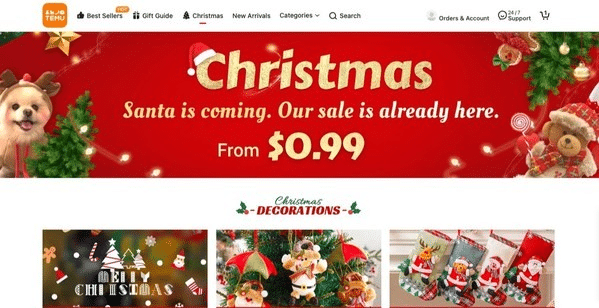The image depicts a detailed screenshot of the T-Mobile website's Christmas-themed section. 

In the top left corner, the T-Mobile logo, distinctively orange, is clearly visible. Adjacent to the logo are navigational tabs labeled Bestsellers, Gift Guide, Christmas, New Arrivals, Categories, and a search icon represented by a magnifying glass. 

On the top right, icons for profile access (orders and account), 24/7 support, and a shopping cart with a notification showing one item are neatly arranged.

Currently active is the Christmas tab, featuring a festive banner; the word “Christmas” prominently displayed with a Santa hat adorning the letter "C." The banner cheerfully proclaims, "Santa is coming. Our sales are already here from 99 cents," accompanied by charming images: a dog wearing reindeer antlers, decorated Christmas trees, a star, gingerbread figures, bow ties, and a bear dressed in a Christmas hat and scarf while holding a lollipop.

Below the main banner, three smaller banners showcase Christmas decorations. The first banner reads "Merry Christmas," adorned with candy canes, Christmas trees, and Santa Claus imagery. The central banner highlights a Christmas tree festooned with ornaments, featuring a snowman, Santa Claus figures, and gingerbread men. The third banner presents a festive collection of stockings, depicting Santa Claus, a playful dog, a reindeer, and various other cheerful holiday symbols. 

Overall, the screenshot effectively captures T-Mobile's festive spirit and promotional enthusiasm for the holiday season.